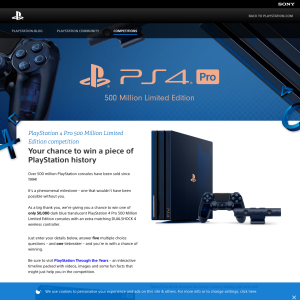The advertisement for the PlayStation 4 is a compact, visually-striking square, featuring key information arranged within various colored banners and sections. At the top, a black banner hosts some text in the top right and a white icon on the left, both too small to read. To the right of the icon, there is additional grayish text also too small to decipher. Below this, three more pieces of information, equally minuscule, are present in a subsequent line.

Occupying about a fourth of the advertisement, the center section is set against a vibrant blue background. Prominently displayed are a game controller and the PS4 logo, followed by a smaller square with "Pro" inscribed inside it. This section features a pumpkin-colored design, with the word "Pro" rendered in blue.

Underneath, bold text states, "500 Million Limited Edition." Further down, a depiction of the PlayStation Pro from a rear view is accompanied by the text, "PlayStation Pro 500 Million Limited Edition Competition." This is coupled with an enticing line, "This Is Your Chance to Win a Piece of PlayStation History." The remaining text is too small to interpret.

The bottom of the ad is capped off by a slim blue banner, adding a cohesive finish to the overall layout.